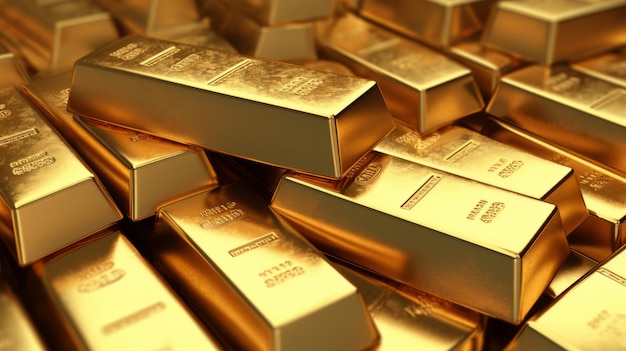The photograph showcases a large stack of gold bars, arranged in a somewhat haphazard manner, with some bars precariously angled and partially sliding between one another. The pile appears to consist of dozens, if not hundreds, of identical gold bars. These bars exhibit a polished, shiny exterior, particularly more reflective on their tops compared to their sides. Each gold bar bears engraved text, though the blurriness of the image prevents the text from being legible. Notably, one gold bar, located slightly higher up and towards the center left of the stack, is scratched on its surface, likely due to other bars sliding over it. The lighting in the image accentuates the scratches and the overall reflective quality of the gold bars, giving them a luminous appearance.